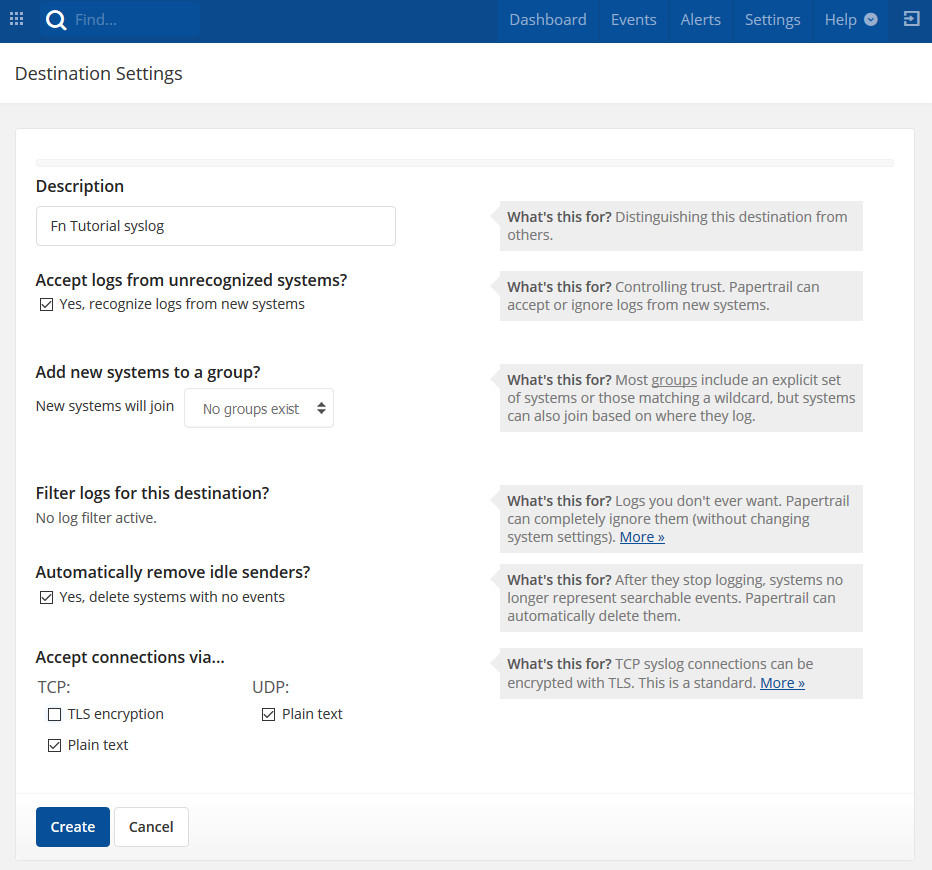This image, sourced from a website, features the "Destination Settings" interface. At the top, a blue rectangle spans the width of the image, housing a white search icon accompanied by the prompt 'find...'. To the right within the same blue bar, navigation options include "Dashboard," "Events," "Alerts," "Settings," and "Help." Below this top section, the middle area of the image showcases a gray square overlaid with a larger white square, exposing only a sliver of the gray background.

The content within the white square begins with the title "Description" followed by several configuration options. The text reads "Fry Tutorial Scythe Log" and lists various log acceptance settings:
- "Accept logs from unrecognized systems" with a checked option to "Yes, recognize logs from new systems."
- "Add new system to a group," indicating that "new systems will join."
- "Filter logs for this destination" with an option to "automatically remove idle senders," followed by "Yes, delete systems with no events."

At the bottom of this section, the text "accept connection via" appears alongside selectable options including "TCP," "UDP," and "plain text."